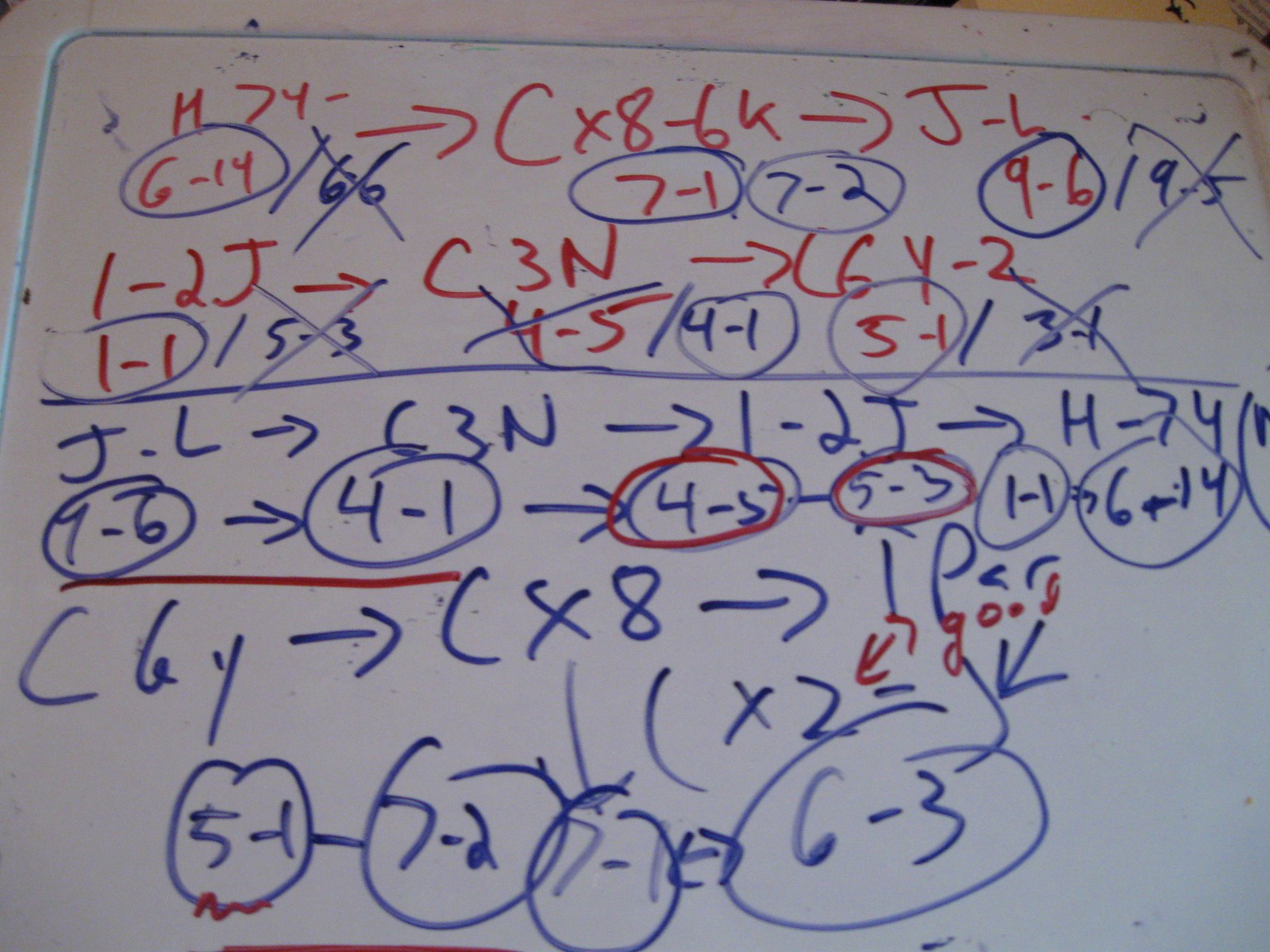This is a color photograph showcasing a white dry erase board densely covered with various mathematical equations, numbers, and letters. The equations span across the board with numerous annotations and alterations. Here is a detailed breakdown of the inscriptions:

- At the top left, it starts with "H7 4 - 6 - 14 / 66", with "66" crossed out.
- An arrow points right to the next equation: "C × 8 - 6K".
- Another arrow points right to "J - L".
- Below that, sequences such as "7 - 1", "7 - 2", "9 - 6" are circled. 
- "19 - 5" is crossed out, followed by "1 - 2J".
- An arrow points right to "C3N".
- Another arrow directs to "6Y - 2".
- Below that, "1 - 1" is circled, with "15 - 3" and "4 - 5" crossed out.
- The sequence "4 - 1" and "5 - 1" are circled followed by a diagonal line and "3 - 1" crossed out.
- "J - L" is written again with an arrow leading to "63N".
- Another arrow points to "1 - 2J".
- This sequence continues with "H - 7, 4", "7 - 6" circled, and an arrow leading to "4 - 1" circled.
- Another arrow points to "4 - 5" and "5 - 3" circled, followed by "1 - 1" circled.
- The sequence "6 + 14" is circled with "C 6 Y" next to it.
- An arrow points to "C × X", and another points to "1 P A R × 2".
- Next to this, in red writing, the word "good" is written.
- Additional circled sequences include "5 - 1", "7 - 2", and "7 - 1".
- A double-sided arrow connects "6 - 3".

The board is a chaotic yet methodical presentation of a complex mathematical or logical problem, punctuated with circled figures, crossed-out components, and guiding arrows to possible solutions or next steps.